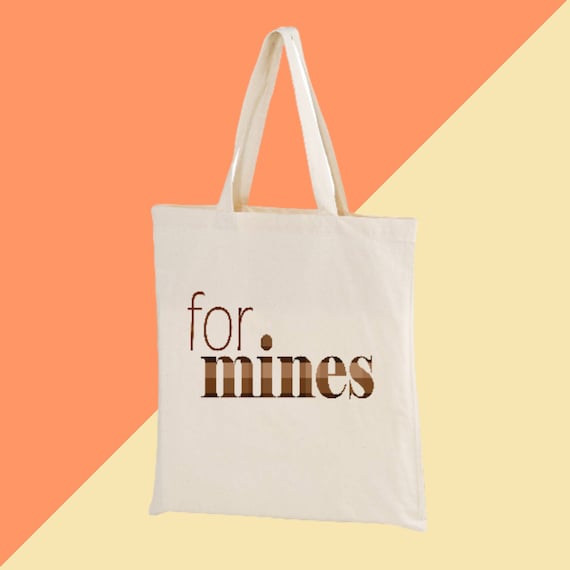The image features a centrally positioned, plain white canvas tote bag with straps that appear to be held upright, as if hanging on an invisible peg. The tote bag prominently displays the text "Four Minds," where "Four" is offset slightly above the "M" in "Minds." The word "Minds" features a gradient color band ranging from light brown to dark brown.

The background is split diagonally, forming two connected triangles, which together create a square. The top triangle is a peach color, while the bottom triangle is a light tan pastel hue. Overall, the color palette includes shades of orange, yellow, tan, and multiple browns, contributing to a visually warm but minimalistic aesthetic.

The tote bag is the sole object in the image, which suggests it might be a stock photo intended for use on a website or in a catalog for marketing purposes. The absence of any other elements or people emphasizes the product itself, making it the focal point of this simple yet sophisticated composition.